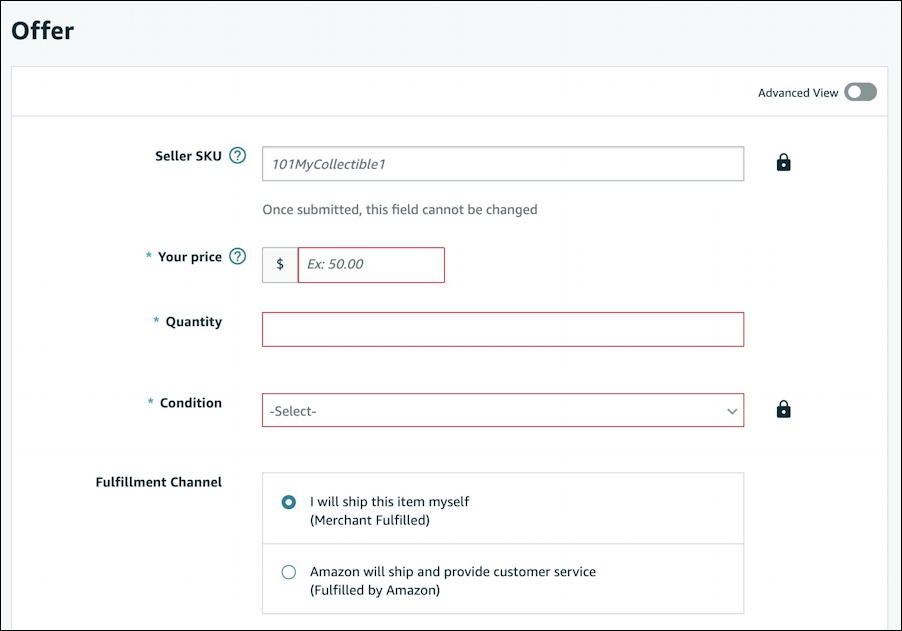This landscape-format, color image is a detailed screenshot captured from a laptop or computer. The image focuses on a functional and straightforward window titled "Offer." This window appears to be a form for submitting an offer for a product. The form is neither particularly designed for aesthetic appeal nor sleek but prioritizes functionality.

The first field labeled "Seller SKU" indicates an example entry "101 My Collectible One," which seems to be the username or the unique identifier for the seller. Following this, there is a field where the user can insert their price, with an example value set at $50. Users have the flexibility to choose their preferred currency by clicking on the dollar sign button, which likely reveals other currency options such as pounds.

Next, the form requires the user to fill out a text box specifying the quantity of the product they are offering. Following the quantity field, there's a selection list for the condition of the item, which, although the options aren't visible, presumably includes choices like "New," "Like New," and "Good Condition."

The final section of the form is dedicated to fulfillment channel options, offering two choices: "I will ship this item myself" and "Amazon will ship and provide customer service."

Overall, the screenshot meticulously captures each interactive element of the "Offer" window, detailing how a user can input and select various pieces of information to create a product offer.